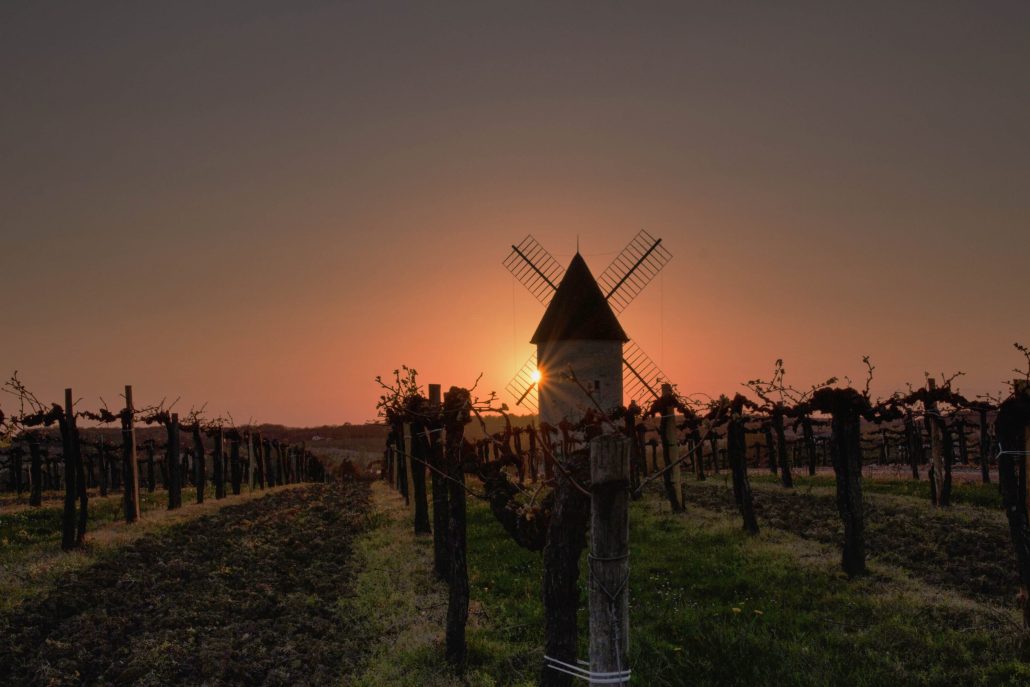This detailed outdoor photograph captures a serene vineyard at either sunrise or sunset, characterized by a soft, somber mood with dark tones. The sun is delicately perched on the horizon, casting an orangish-purple hue in the sky, partially obscured behind a classic Dutch-style white windmill with a dark conical roof and four large blades visible, standing like an "X." In the medium background, a window is subtly present near the windmill, adding to the rustic charm of the scene. The foreground is dominated by rows of grapevines extending into the distance, their posts connected by wire, with green grass growing between the rows. The grapevines are mostly withered, hinting that the photograph was taken outside of the harvest season. The colors transition beautifully from muted browns and greens in the foreground to a pale peach near the horizon and gradient grays in the sky above, creating a photorealistic representation of a quiet, ancient vineyard landscape that evokes a sense of tranquility and timelessness.